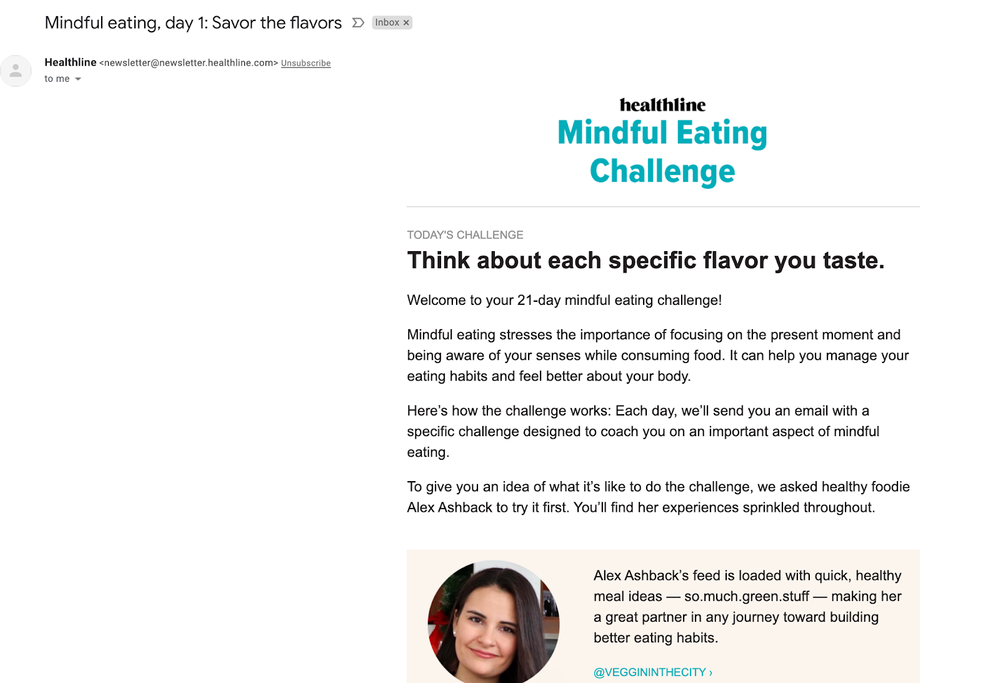**Detailed Caption:**

The image features a layout promoting a "Mindful Eating Challenge." On the top left, "Mindful Eating Day" is prominently displayed. Beneath it, a subtitle reads "Mindful Eating, Day One: Savor the Flavors," accompanied by an arrow pointing to the right. To its right, a gray rectangle labeled "Inbox" with a 'K' symbol next to it and a light gray circle with a person icon complete the section.

On the right-hand side, the word "Headline" appears, followed by "Mindful Eating Challenge" in blue text. Below a gray line, instructions are given: "Today's Challenge: Think about each specific flavor you taste."

Accompanying the challenge greeting is an introduction: "Welcome to your 20-day Mindful Eating Challenge! Mindful eating emphasizes focusing on the present moment and being aware of your senses while consuming food. It can help you manage your eating habits and feel better about your body. Here's how the challenge works: Each day, we'll send you an email with a specific challenge designed to coach you on an important aspect of mindful eating. To give you an idea of what it's like to do the challenge, we asked healthy foodie Alex Ashback to try it first. You'll find her experience sprinkled throughout."

At the bottom, a peach-colored rectangle features a circular image of a woman's face. It is labeled "Alex Ashback's feed is loaded with quick, healthy meal ideas – so much green stuff – making her a great partner in any journey towards building better eating habits." It also includes the handle "@veggieinthecity" in green text.